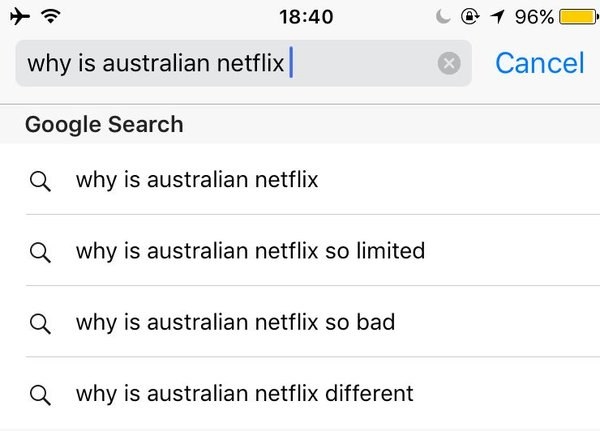**Screenshot Description:**

The screenshot captures a webpage displayed on a tablet or smartphone, featuring various interface elements. Dominating the upper section, on the left side, a black airplane silhouette, indicative of airplane mode, is positioned next to a black Wi-Fi symbol. Centrally displayed, the time is set at 18:40 in military format. Adjacent to this, a gray crescent moon suggests a night mode setting. 

Further to the right, a black circle housing a black lock icon hints at a privacy mode, while a right-facing arrow, also black, precedes a yellow battery icon indicating a 96% charge. 

Below this status bar, a gray search bar features black text, "why is australian netflix," with a blue cursor marking the text input position. Positioned on the right edge of the bar is a dark gray circle with a white "X," serving as a clear button. In cyan blue, the word "Cancel" is clearly visible to the right of the search bar.

Beneath the search bar, a lighter gray rectangle with bold black text reading "Google Search" is highlighted by a series of magnifying glass icons on the left. These icons precede auto-suggested search queries, each separated by thin gray lines and rendered in regular black text:

1. Why is Australian Netflix Australian Netflix
2. Why is Australian Netflix so limited?
3. Why is Australian Netflix so bad?
4. Why is Australian Netflix different?

These suggestions dynamically complete based on the user's typed input. The interface elements collectively suggest the device is in airplane mode, actively searching on Google with auto-suggestions visible.